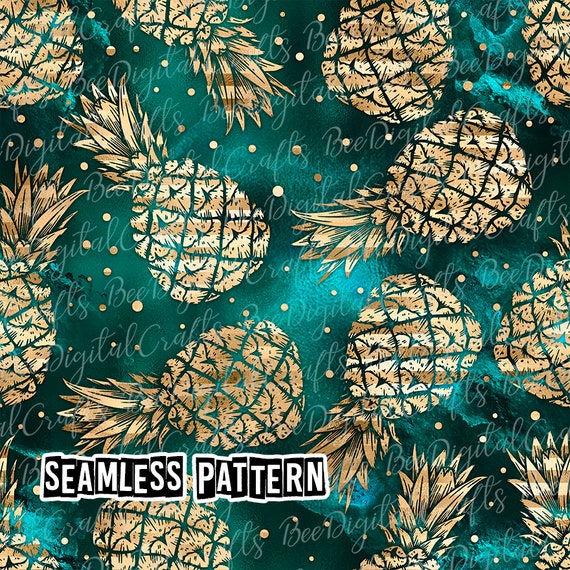The image showcases a seamless pattern predominantly featuring golden pineapples, each identical in design but oriented differently, distributed across a greenish-turquoise background. Small golden-brown dots pepper the background, matching the color of the pineapples. Over the entire image, a transparent watermark repeatedly displays the text "B digital crafts," implying a connection to the company, possibly specializing in digital design assets. In the bottom left corner, the words "seamless pattern" are clearly visible within a white box with a black outline. The image resembles a blanket or fabric design, seamlessly integrating the pineapples and the text.